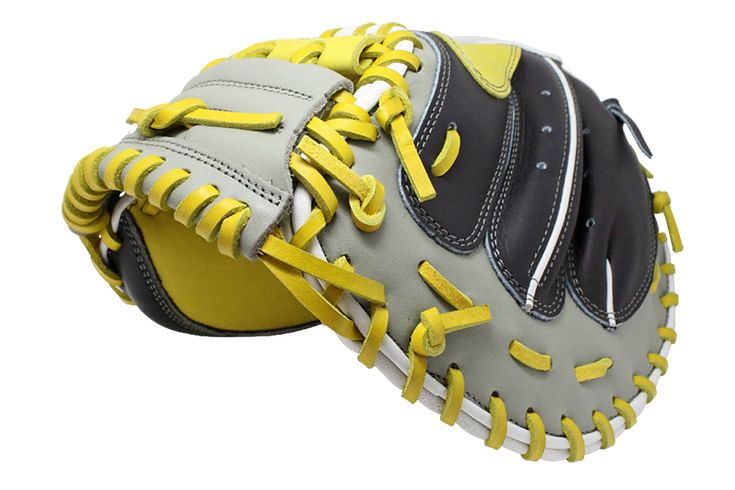The image showcases a baseball catcher's mitt set against a plain white background. The glove features a striking design with a shiny silver top portion and a prominent black section adorned with white stripes on the finger area. Yellow stitching outlines the exterior and extends to the interior near the thumb section. A yellow patch with black stitching is also present, adding visual interest. The interior of the mitt is predominantly yellow, with some black leather sections stitched together using white thread. The middle finger area includes three air vents for breathability. Overall, the glove, with its intricate weaving of thick yellow leather and robust construction, appears to be exceptionally well-made.